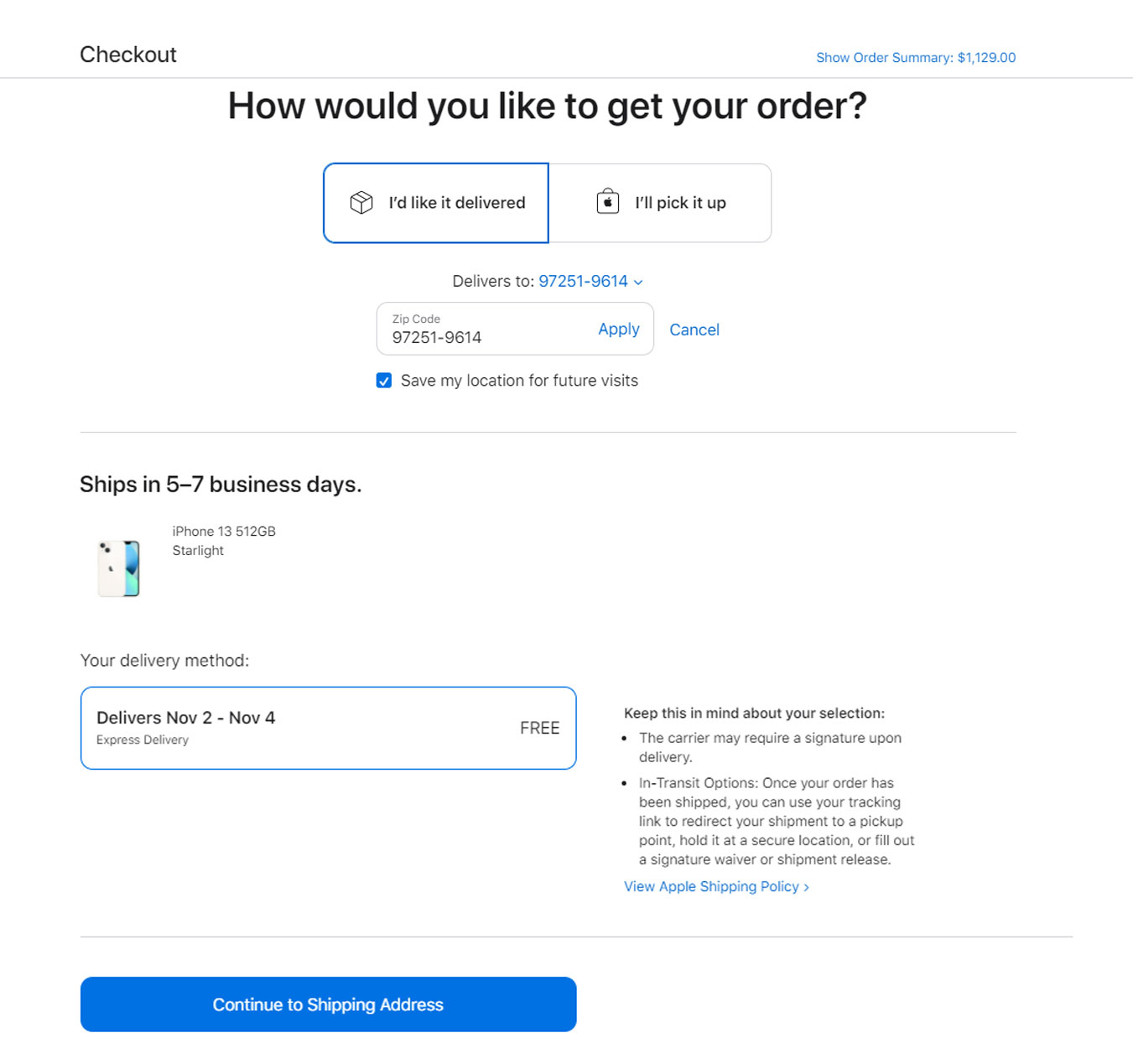The screenshot displays a detailed view of a checkout page for an item that has been ordered online. 

**Header Section:**
- **Top Left Corner:** The word "Checkout" is prominently displayed.
- **Top Right Corner:** There's an option labeled "Show Order Summary," accompanied by the total amount of $1,129.00.

**Main Content:**
- **Delivery Options:**
  - **Primary Question:** "How would you like to get your order?"
  - **First Option:** "I'd like it delivered." This choice is highlighted with a blue border.
  - **Second Option:** "I'll pick it up." This option remains unbordered.

- **Delivery Address:**
  - Stated delivery to zip code: 97251-9614.
  - A field displaying the same zip code, labeled "Zip Code."
  - An option to save this location for future visits, indicated by a checked box labeled, "Save my location for future visits."
  - Additional information states that shipping will occur within 5-7 days.

**Product Details:**
- **Product Icon:** An image of an iPhone.
- **Product Description:** "iPhone 13, 512GB Starlight."

**Delivery Method:**
- A defined section titled "Your Delivery Method" featuring a bordered rectangle with the text, "Delivers November 2-4 Express Delivery Free." This section is highlighted with a blue border.

- **Important Notice:** On the right, a reminder states, "Keep this in mind about your selection. The carrier may require a signature upon delivery."

**In Transit Options:**
- An informative section that explains users can redirect their shipment to a pickup point, hold it at a secure location, or opt for a signature waiver or shipment release using the tracking link once the order has been shipped.
- A link to "View Apple Shipping Policy" is provided.

**Footer Section:**
- A prominent blue rectangle button with centered white text reads, "Continue to Shipping Address," encouraging the user to proceed with the next step in the checkout process.